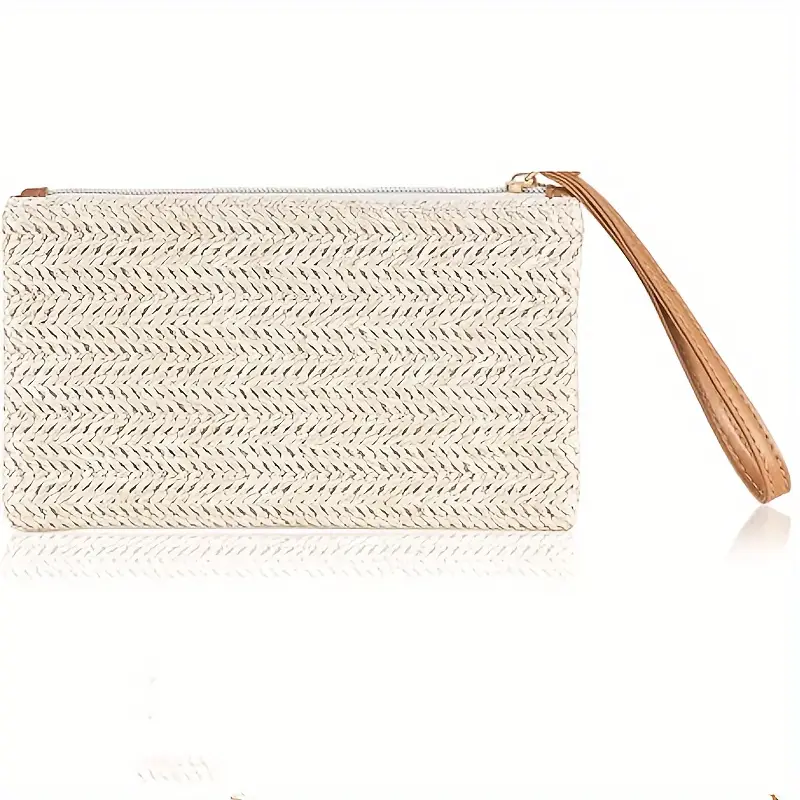The image captures a close-up of a small, rectangular purse or wallet placed on a highly reflective white surface, creating subtle reflections of both the purse and its strap. The purse features a distinct, textured exterior made of a material that alternates between a cream or off-white hue interspersed with thin, black, diagonal lines resembling zigzags or tire tread marks. This gives it an intricate, patterned appearance. The top of the purse is secured with a white zipper, which is predominantly closed, revealing a small brown leather tab at the zipper's starting point. On the opposite end, the zipper is accented by a gold piece connected to a light tan to brown leather strap. This strap is slim enough to be worn around the wrist and hangs down delicately from the purse's side. The background is stark white, emphasizing the purse's elegant and minimalistic design.